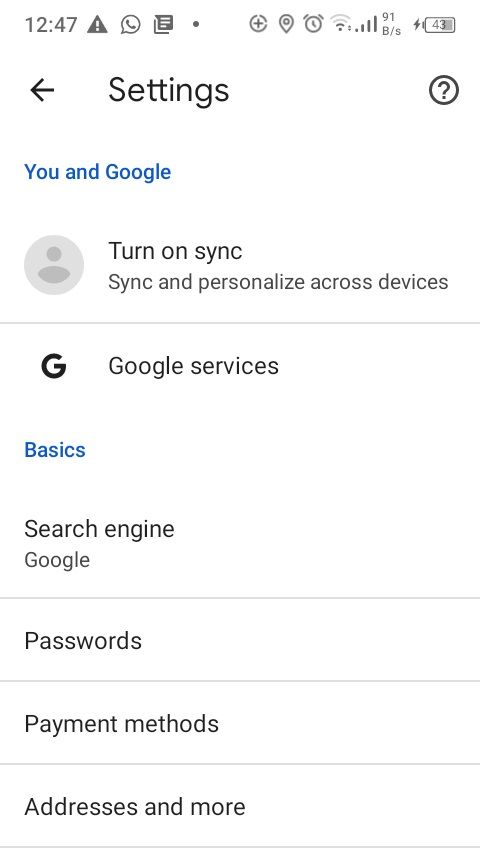Screenshot of a mobile phone in portrait orientation displaying the settings menu. The screen has a white background and is topped by a status bar that shows the time at 12:47, with various icons indicating phone status, including a battery symbol at 43%. Below this status bar are navigational elements: a back arrow on the left and the word "Settings" prominently featured in the center, with a question mark inside a circle on the right.

Further down, a blue section labeled "You and Google" appears, featuring an icon of a person on the left and an invitation to "Turn on sync," followed by the description "Sync and personalize across devices." Below this, a thin gray divider line separates it from a "G" icon labeled "Google services."

The next section, titled "Basics" in blue, lists several options: 
- "Search engine," with "Google" written underneath it.
- "Passwords," with a gray line beneath it.
- "Payment methods," also followed by a gray line.
- "Addresses and more," separated by yet another gray line.

The entire settings menu uses a consistent black font, and densely packed with pertinent information and options for managing Google services and personal device settings. The background remains stark white, providing a clean and structured presentation that is very straightforward and easy to navigate.